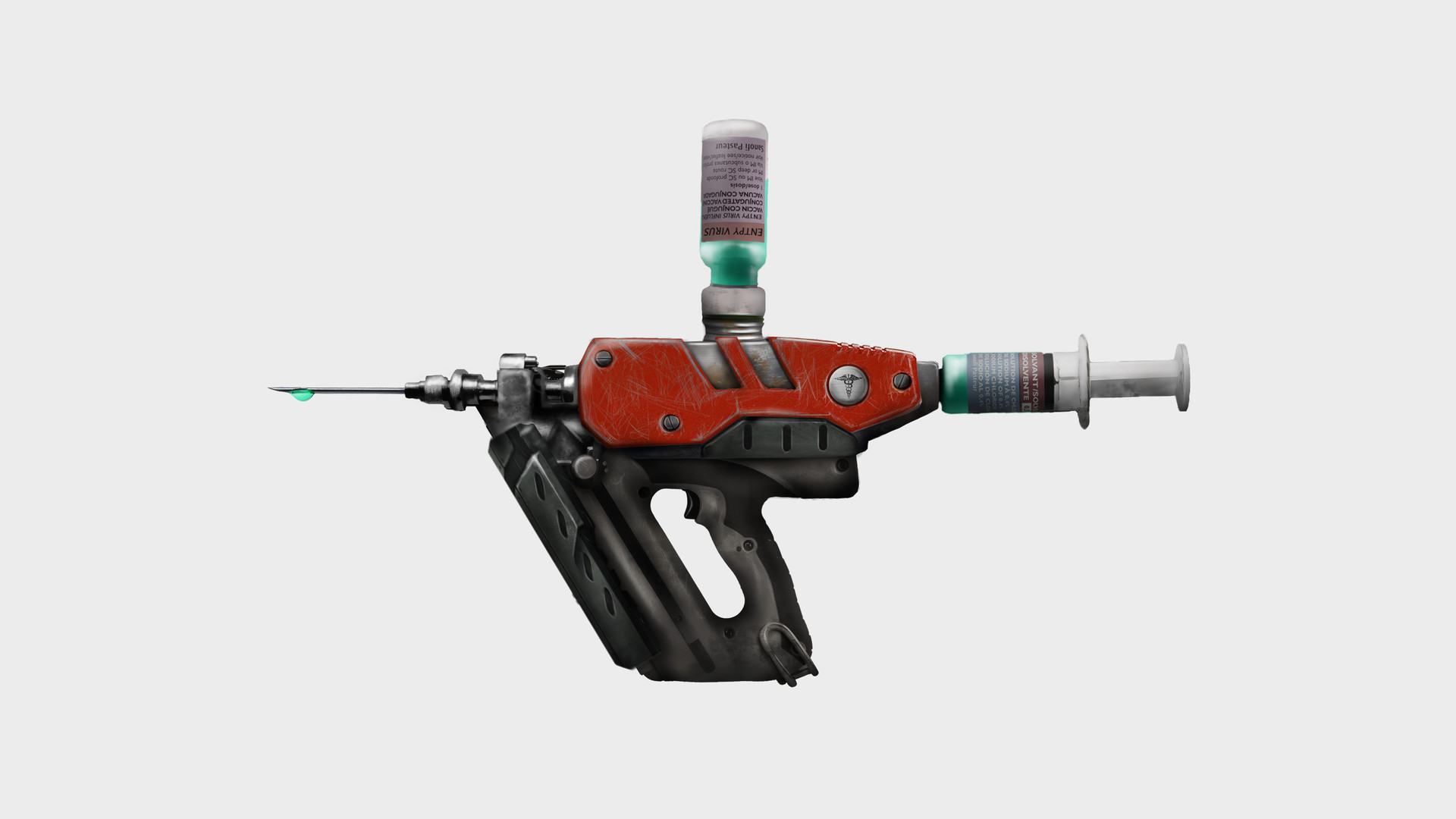This digital image depicts a weapon or medical device reminiscent of props from video games or cartoons. The device, resembling a handheld drill or gas pump handle, features a gun-like form with a prominent syringe needle at its tip. Instead of bullets, the device administers a liquid substance. The rear handle is styled after a syringe plunger, facilitating the dispensing action. 

Atop the device, an inverted glass vial filled with blue or green medicine is securely attached, simulating the process of drawing medication like in a clinical setting. The vial’s position allows the liquid to flow directly into the device, which is accented with black, red, and silver hues. A noticeable drop of the medicine is visible at the needle's tip, highlighting its purpose for injections. The composition and vibrant coloring underscore the dual nature of this imaginative tool-slash-weapon, which merges the aesthetic of medical and combat equipment.